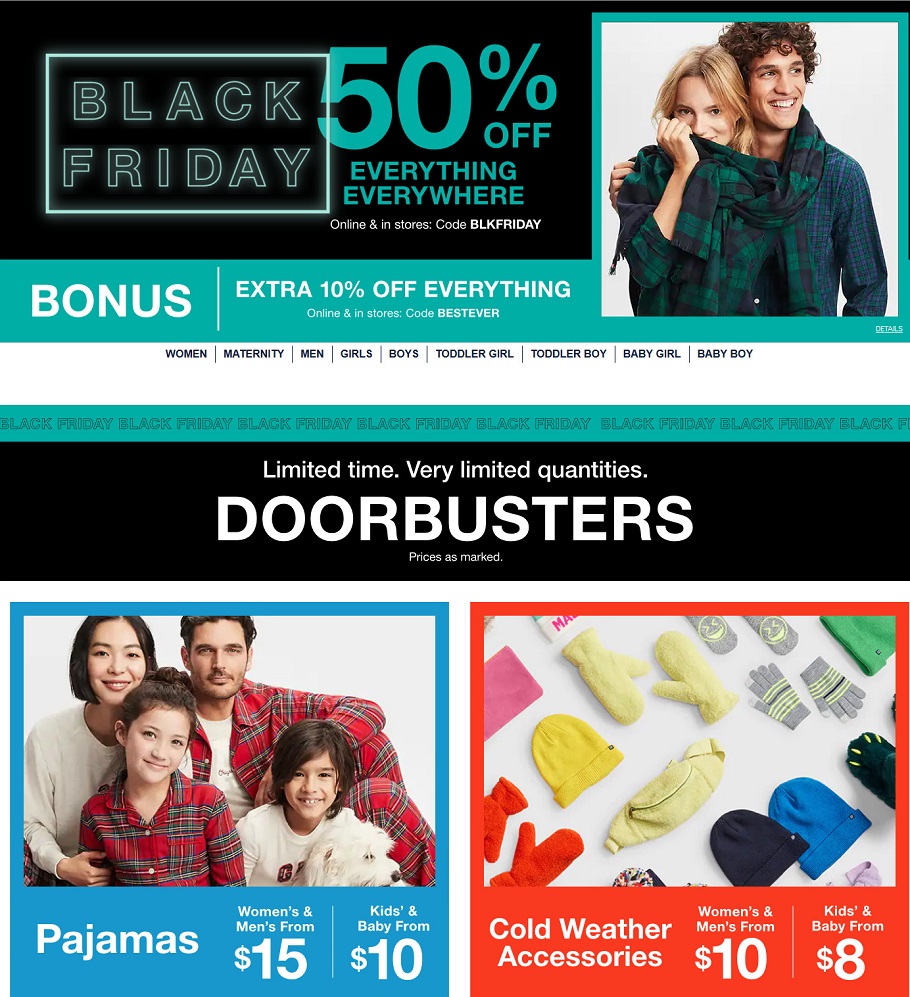The image is a screenshot of a retail store's website, prominently displaying their Black Friday deals. At the top of the page, a large black banner with mint-colored text announces "50% off everything, everywhere, online and in stores" for Black Friday. To the right, there is a stock image of a man and a woman modeling flannel clothing. 

Beneath this, a mint-colored border highlights an additional offer, stating "Bonus: Extra 10% off everything online and in stores" with the label "Best Ever." Moving down, the website's menu bar is displayed against a white background, featuring various options for different categories: Women, Maternity, Men, Boys, Girls, Toddler Girl, Toddler Boy, Baby Girl, and Baby Boy. 

A repetitive teal banner runs vertically down the screen, persistently proclaiming "Black Friday, Black Friday." Below this, another black banner alerts visitors about a special, time-sensitive deal with "Limited time, very limited quantity, door busters, prices as marked."

At the bottom of the page, two more promotional blocks are displayed. The left block, in blue, advertises pajamas with a stock image of a family (mother, father, son, and daughter) all dressed in pajamas, offering women's and men's pajamas for $15 and kids' and babies' pajamas for $10. The right block, in red, focuses on winter accessories, showcasing various items and offering women's accessories for $10 and kids' and babies' accessories for $8.